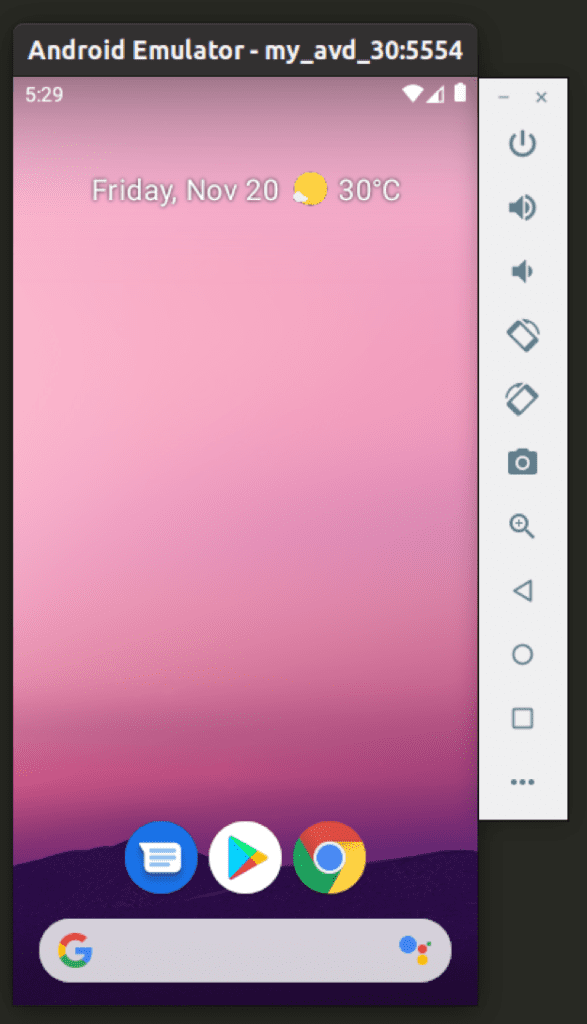The image depicts an Android emulator interface, specifically labeled as "Android Emulator - my_AVD_30:5554" at the top of the screen. The time displayed on the emulator is 5:29, located at the top left corner. To the top right, there is a fully filled battery icon, indicating a full charge, alongside a signal strength icon with one bar missing, and a fully filled Wi-Fi signal strength icon.

In the top center of the screen, the date is displayed as "Friday, November 20th," and the temperature is shown as 30 degrees Celsius. An icon of a sun partially obscured by a small white cloud accompanies the temperature reading.

Moving to the bottom middle of the screen, there are three app icons. The first is a text messaging app with a blue background, followed by the Google Play Store app, and then the Chrome browser app. Beneath these icons lies a Google search bar.

On the right side of the screen is a vertical array of icons: a power button icon at the top, followed by volume control icons, screen rotation icons, and a camera icon towards the bottom.